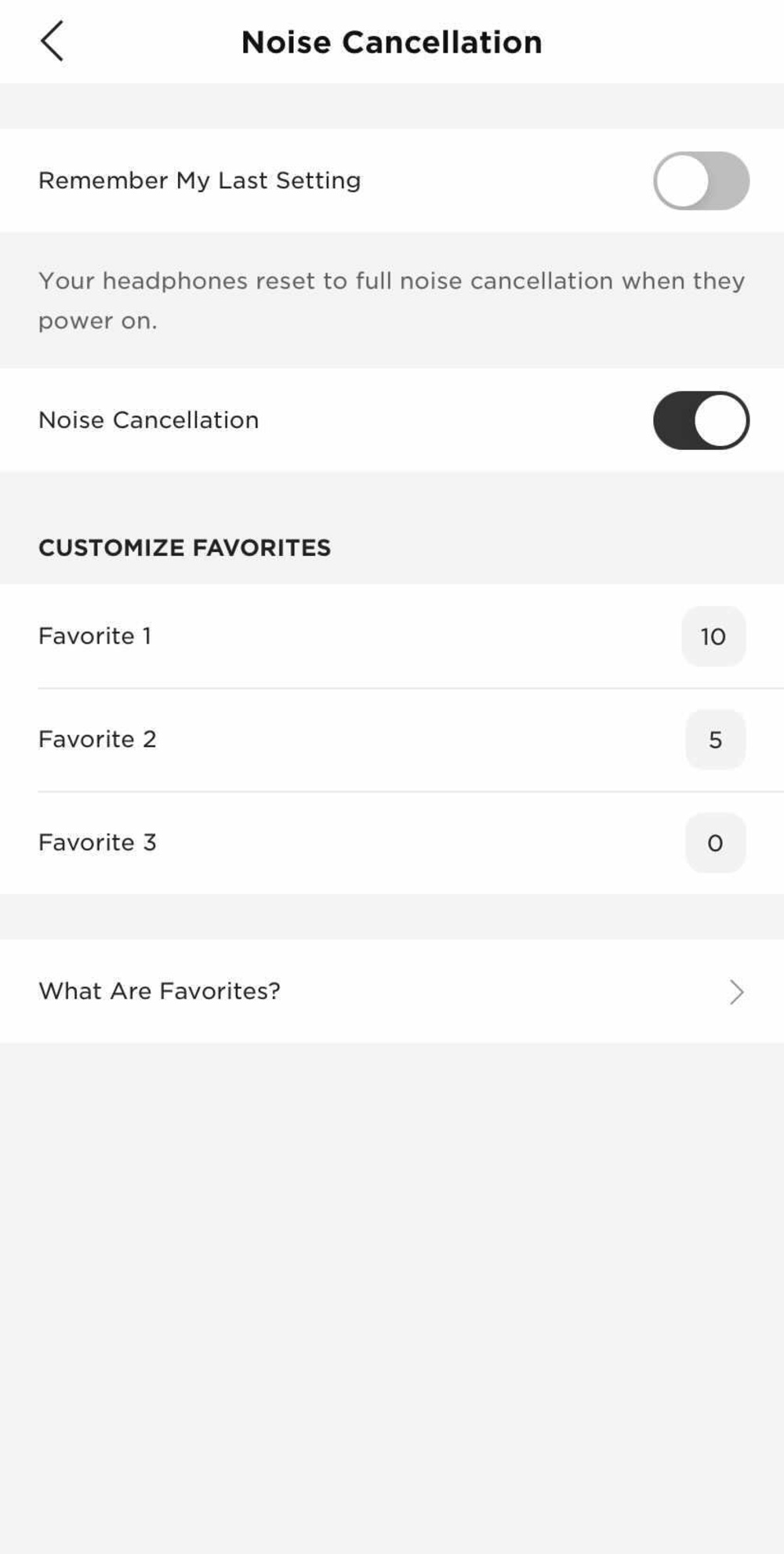The image showcases a part of a cell phone screen featuring settings for noise cancellation. The background alternates between white and gray sections, creating a structured layout. 

At the top of the screen, the title "Noise Cancellation" is displayed in black text, accompanied by a left-facing arrow. Below this, a thin gray strip separates the sections.

Next, the "Remember My Last Setting" option is listed on a white background and is toggled off. Beneath this, there's an explanatory note stating, "Your headphones reset to full noise cancellation when they power on."

The following section, "Noise Cancellation," is currently toggled on. Underneath, the section "Customized Favorites" is highlighted in black text.

The customizable settings include:
- Favorite One: 10
- Favorite Two: 5
- Favorite Three: 0

Each favorite option is displayed with a white background, and the numerical values are housed in gray squares aligned on the right side of the screen.

Further down, there is a section titled "What are Favorites?" with a small right-facing arrow at the extreme right. The bottom half of the image features a solid gray background, concluding the layout.